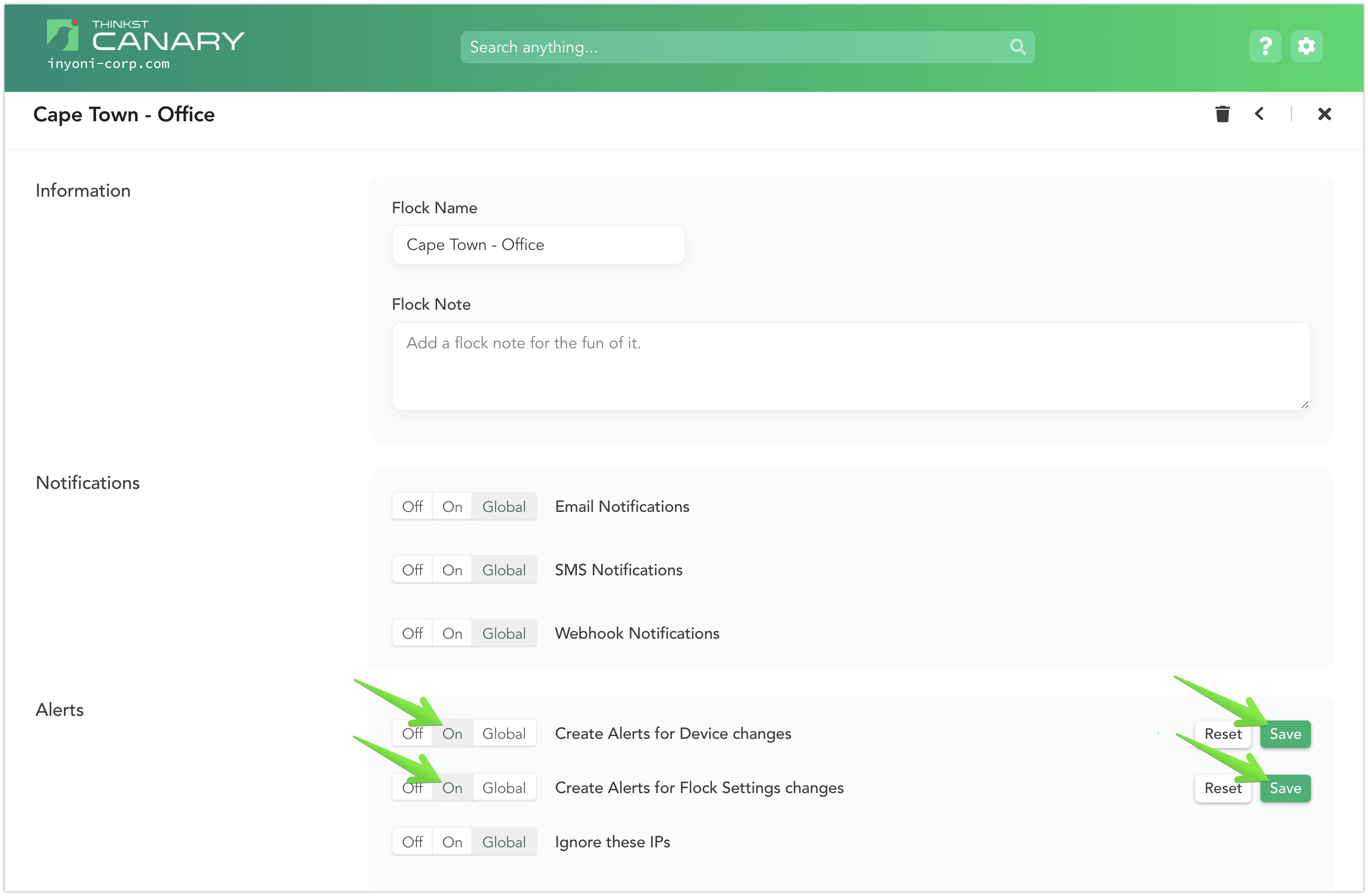The image is a screenshot from the Canary website, which features a vibrant green header section, with the rest of the page predominantly in white. The website's logo includes a green canary bird icon. At the top of the page, there is a search bar with the placeholder text "Search anything," accompanied by a question mark icon for help and a gear icon for settings.

Further down, the header displays the title "Cape Town-Office" alongside the label "Information" and the flock name "Cape Town-Office." There is a section for adding flock notes, indicated by the prompt "Add a flock note for the fun of it."

The notification settings are prominently featured, with options to toggle notifications on and off. There are three types of notifications available: Email Notifications, SMS Notifications, and Webhook Notifications. Each type has its own toggle switch and global settings.

Towards the bottom of the screenshot, there is an alerts section with similar on/off toggle switches and global settings. Digital green arrows have been added to the image, highlighting the "On" switches and pointing towards two green buttons labeled "Save," indicating critical interactive elements. The page also includes options for users to "Reset" or "Save" their settings.